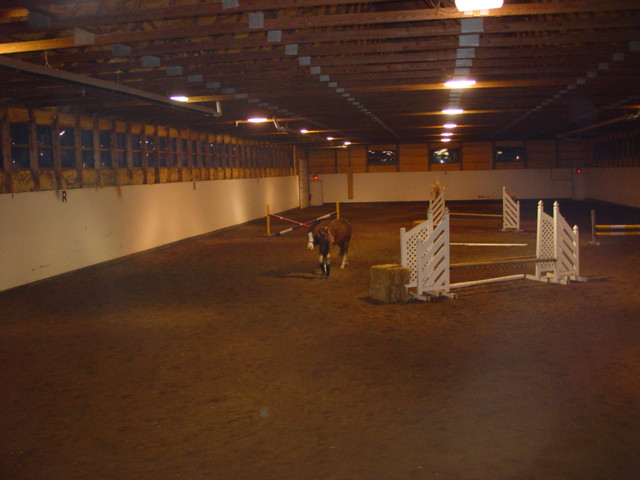The photograph captures a large indoor horse arena at night, with lights casting a warm glow from the ceiling, illuminating the scene. The ceiling is lined with horizontal wooden cross beams, each adorned with silver markings spaced at regular intervals. Suspended down the center, between every few beams, are powerful lights that brighten the arena.

In the midground, a brown horse with distinct white markings on its face and feet stands almost centrally, its head slightly tilted forward. A woman with long blonde hair stands in front of the horse, wearing a brown shirt, black shorts, and tall black boots. Her outfit and poised stance suggest she is the rider.

Surrounding the arena, wooden stalls with numerous windows line the left and back walls. The left wall features approximately 20 neatly divided windows with a white wall beneath. Similarly, the back wall displays three aligned windows against a brown background. The floor of the arena consists of dark brown dirt, suggesting an area prepared for training.

Scattered around the arena are several practice obstacles for horse jumping. These include three white barriers with crossbars and simpler units, one forming an X shape, placed strategically around the space. The photograph encapsulates a moment of equestrian training under the arena's sturdy, beam-structured roof that expands uniformly, creating a vast and organized environment for both horse and rider.